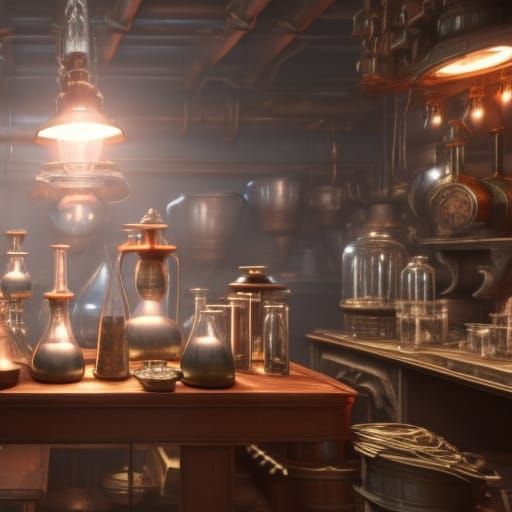This detailed image appears to be a digitally rendered or computer-generated interior of a small, dark room, possibly a kitchen or laboratory, characterized by a distinctly surreal and tidy appearance. The overall color palette is primarily gray and brown, lending a foggy and muted atmosphere to the scene. 

On the left side of the image, there is a brown wooden table topped with various glass jars, some containing a shiny, silver-gray substance, while others are empty. Above this table, a metallic lamp hangs from the ceiling, emitting a warm, yellowish light that bathes the environment, yet paradoxically accentuates the gray tone of the walls and surroundings.

Further details reveal the presence of additional containers, including brown jugs or vases, and clear glass hurricanes with rounded tops, each reflecting the ambient light. To the right, another side table hosts more of these oddly shaped glass jars and containers. 

The background features a grayish wall adorned with silver, vessel-like objects, enhancing the room's laboratory feel. Overhead, the ceiling is lined with visible pipes, adding to the industrial ambiance. Despite the bright glow from the lamps, the room maintains a dim, somewhat eerie quality, emphasizing its likely staged or virtual origin, as it seems too meticulously curated and surreal for a real-life setting.